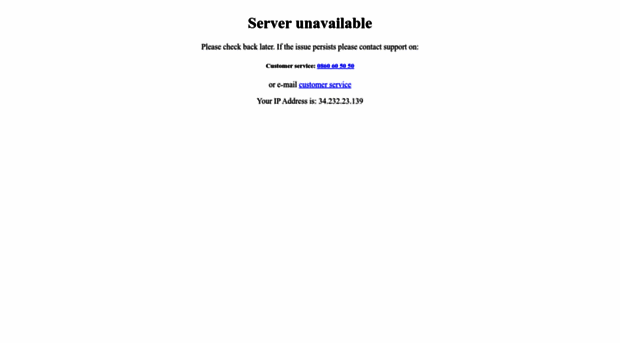The image displays an error message in a bolded, large font that reads "Server Unavailable." Below this message, in slightly smaller text, it states, "Please check back later. If the issue persists, please contact support:" This is followed by a line that reads "Customer Service:" and a non-US formatted phone number, both of which are hyperlinked. The next line reads "Or email" with the text "customer_service" in a hyperlink format. At the bottom, the message "Your IP Address is:" is displayed, followed by an actual IP address. The background of the image is plain white, and all the text is centered on the page, with no additional elements present.